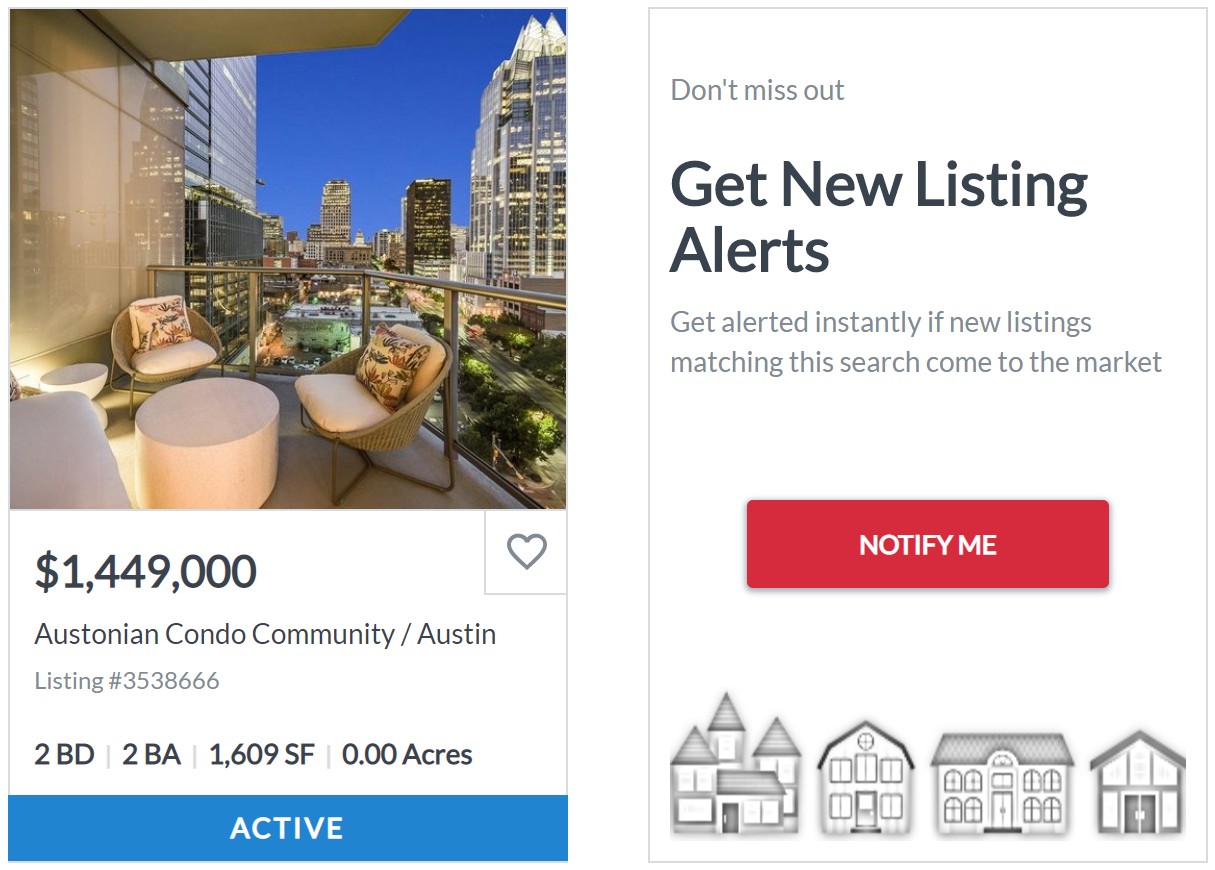This image displays a detailed listing from a Realtor website. On the left side, a large, vivid photograph captures the essence of an upscale Austonian condo community in Austin, Texas. The photo showcases a stunning downtown skyline under a deep blue sky, with a luxurious foreground featuring a well-furnished balcony complete with chairs and a table, highlighting the high-end lifestyle. The listing indicates that the condo is priced at $1,449,000 and offers two bedrooms, two bathrooms, and a living space of 1,609 square feet with no land acreage—as expected for a condominium. The property status is marked as active, with a specific listing number provided. On the right side, there's a prominent box urging potential buyers not to miss out by offering instant alerts for new matching listings, accompanied by a red "Notify me" button for easy sign-up. At the bottom of the webpage, a charming sketch illustrates various house styles, rounding out the visual appeal of the listing.